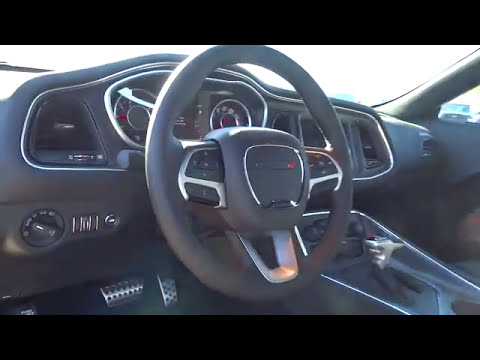The image depicts the interior of a car from the perspective of the driver's seat, focusing closely on the dashboard and steering wheel. The center of the image is dominated by a gray steering wheel, which features various control buttons, including cruise control, on each side. Just behind the wheel, on the dashboard, is a prominent instrument panel with round dials displaying the speedometer and tachometer, outlined in silver.

To the right of the steering wheel, the gear shift box is visible, with a handle for changing gears. The dashboard itself is tall, partially obscuring the windshield, which allows a glimpse of a bright, sunny day outside.

The vehicle's interior is primarily dark gray and black, with accents of silver. Below the dashboard, you can see the silver metal brake and gas pedals. To the left of the instrument panel, a round dial likely controls the headlights, and nearby are the heating switch, headlight switch, fog light switch, and hood release. Vents for heating and cooling are also present on the left side of the dashboard.